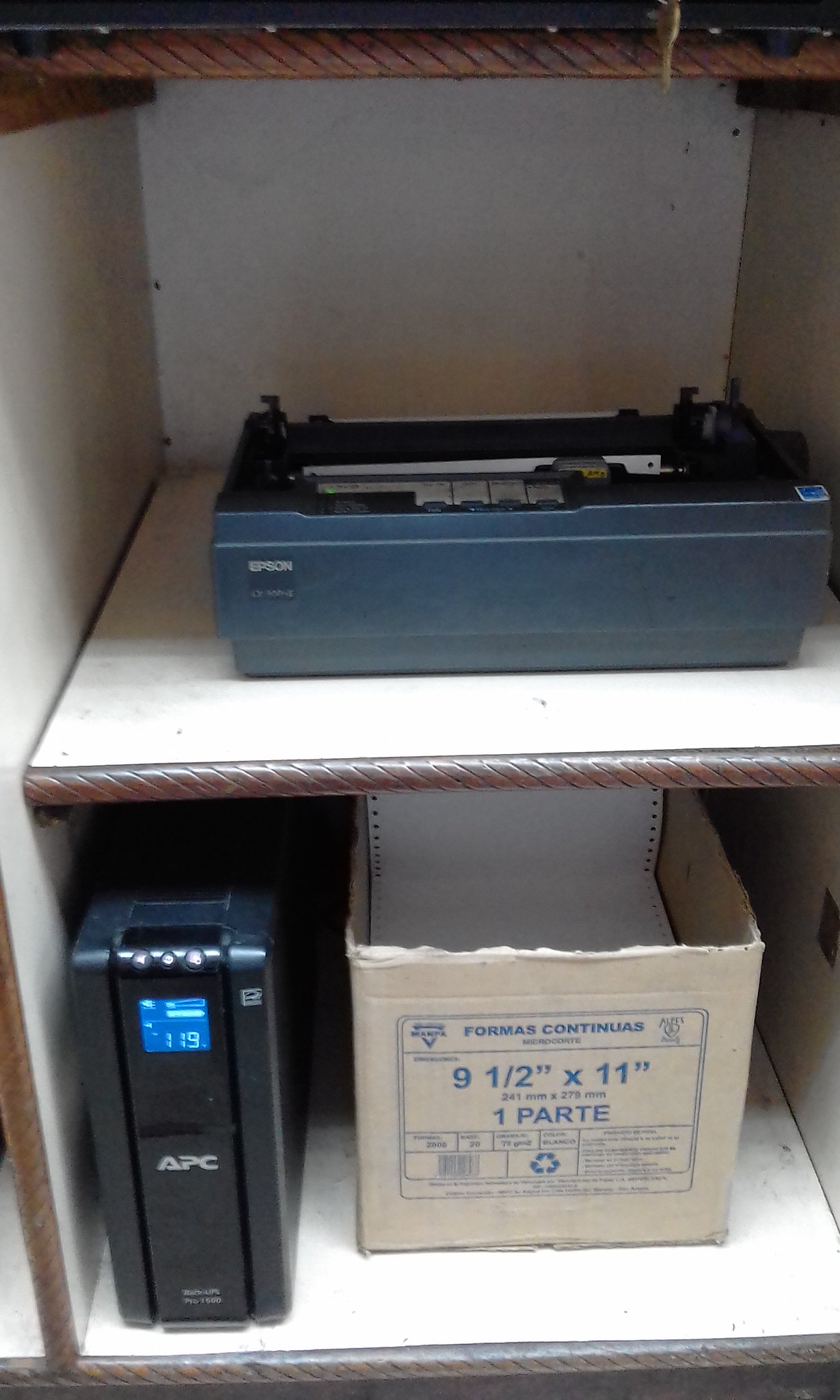This color photograph showcases a somewhat aged and dusty white bookcase or set of open cubby shelves with a silverish or gold edging that varies based on the light. On the top shelf, there is a dark blue Epson printer with distinctive features, including a white bar on top and old-fashioned design elements hinting at its age. The printer stands out due to its dark color against the white shelf background. On the bottom shelf rests a black rectangular machine, marked with the brand APC, featuring an LED display that reads '119'. Adjacent to this machine, also on the bottom shelf, is a white cardboard box with blue lettering that reads "Formas Continuous 9 1⁄2 x 11 1⁄2 inches, one part". This box contains vintage printer paper identifiable by its perforated hole punches on both sides, indicative of continuous feed forms used in older printers.